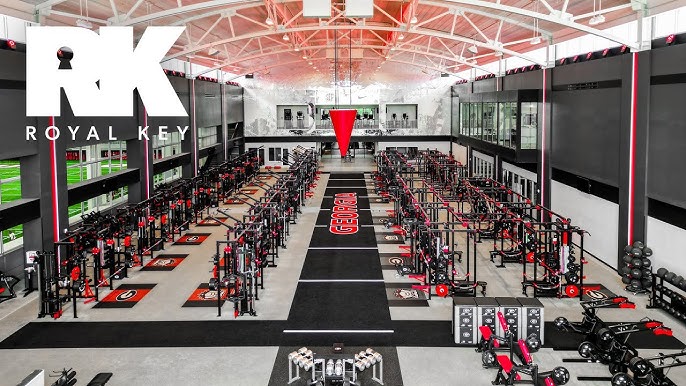The photo depicts the interior of a large, warehouse-like gym situated within a spacious building that spans approximately 200 feet across and stands at least two stories tall. The ceiling is arched, featuring metal support beams that enhance its grandiosity, and is illuminated in a light red hue, contributing to a modern aesthetic. The gym is meticulously organized with rows of various gym equipment, including an abundance of bicycles and weights, suggesting a versatile fitness area. The left wall is painted black, while the right wall has a dark gray upper section and a white lower section. The far wall showcases a distinctive gray and white cloudy print. Dark black columns with red and white stripes are evenly spaced along the side walls. A black pathway or strip runs down the center of the gym, emblazoned with the word "Georgia" in bold red letters. Additionally, at the top left corner of the photo, overlaying the image, is the text "RK" in large white bold letters, with "Royal Key" written in smaller, thin white text beneath it.